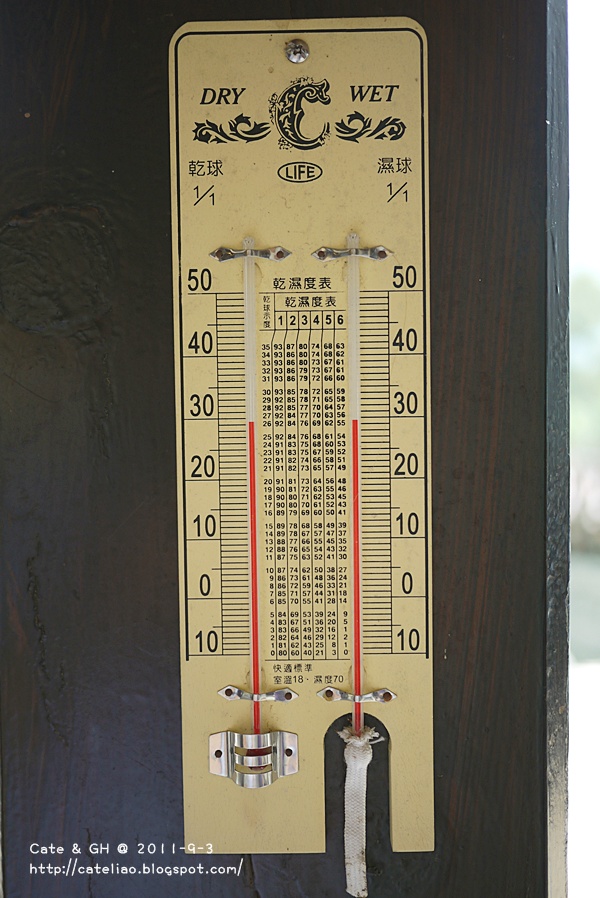This image features a sophisticated thermometer system with distinct components and markings. The system includes two main thermometers encased in a beige-colored rectangular frame, distinguished by an oval, arched cutout at the bottom right. At the top of the frame, the word "DRY" is prominently displayed in bold, uppercase black letters on the left, while "WET" appears correspondingly on the right. A large letter "C" is also visible, accompanied by Asian lettering and the repetitive phrase "1 out of 1."

On the left side of the frame, a transparent tube is securely fastened with a silver bracket system. The tube, marked with numerical increments, starts from 10 and ascends to 50, featuring numerous intermediate markings. The central area of the frame contains additional, less discernible markings. A similar tube is mirrored on the right side, also held in place by a bracket, but this one is connected to a piece of white cloth, suggesting a unique function or measurement process. This tube shares the same numerical markings as its counterpart on the left.

Both thermometers have their red indicators reaching up to approximately the 28-29 mark, nearly touching the 30 line, showing almost identical readings. At the bottom of the frame, there is some writing that includes the names "Kate and GH 2011" along with an indeterminate website, indicating possible creators or a point of reference for this temperature measuring device.